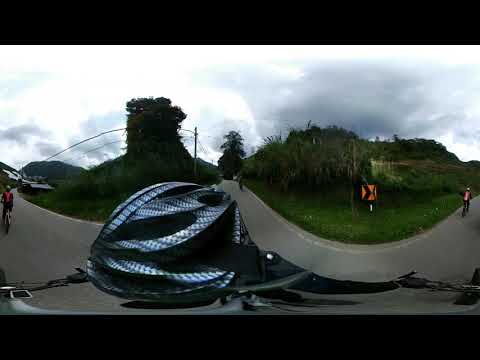This panoramic image, likely taken with a VR or 360 camera, showcases a highly warped perspective reminiscent of fisheye lensing. The primary feature is a curved road that sweeps from the right to the left side of the photo, framed by tall grass, bushes, and intermittent trees. Running through the middle of the image is a curving gray structure, similar to a wall, that arches and dips before ending near the corners.

To the right side of the image, a yellow rectangular road sign with a black arrow is visible along the grassy edge of the road. On the lower half, handlebars and a helmet suggest the viewer's perspective is from a bike rider. A man, possibly walking or running, is faintly visible on the far left. The sky dominates the upper half of the scene, filled with dim, gray clouds that cast a subdued light over the entire landscape. The overall atmosphere of the image is muted and somewhat surreal, highlighted by the blue object with an unclear pattern in the middle and black bars framing the top and bottom.